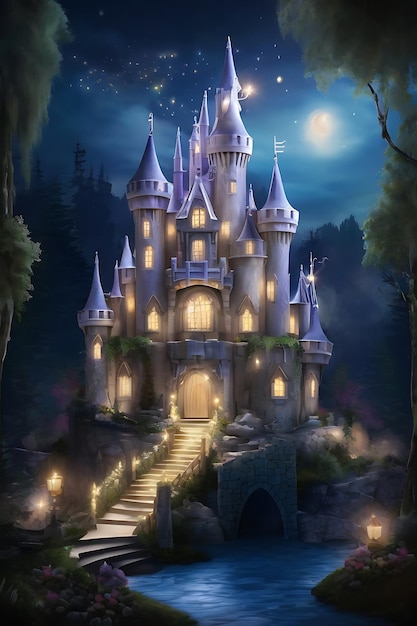This image features a vivid, fantasy-like castle that appears to be an AI-generated or computer-rendered scene. Set against a backdrop of a starry night and a bright full moon, the castle is illuminated with bright electric lights, giving it a welcoming and magical ambiance. The structure is characterized by numerous pointy towers—around twenty spires—that rise sharply into the sky. Accessible only by boat, the castle stands by a flowing blue river or moat, with stone steps leading from the water up to the entrance. These steps, as well as the interior windows, are aglow with a golden light, reminiscent of candles, though the intensity suggests electric lighting. Surrounded by a dense forest with weeping willow trees, and decorated with various flags, the castle combines a medieval essence with modern elements, highlighted by square windows and lit pathways. The moonlight casts a serene glow over the entire scene, enhancing its enchanting quality.